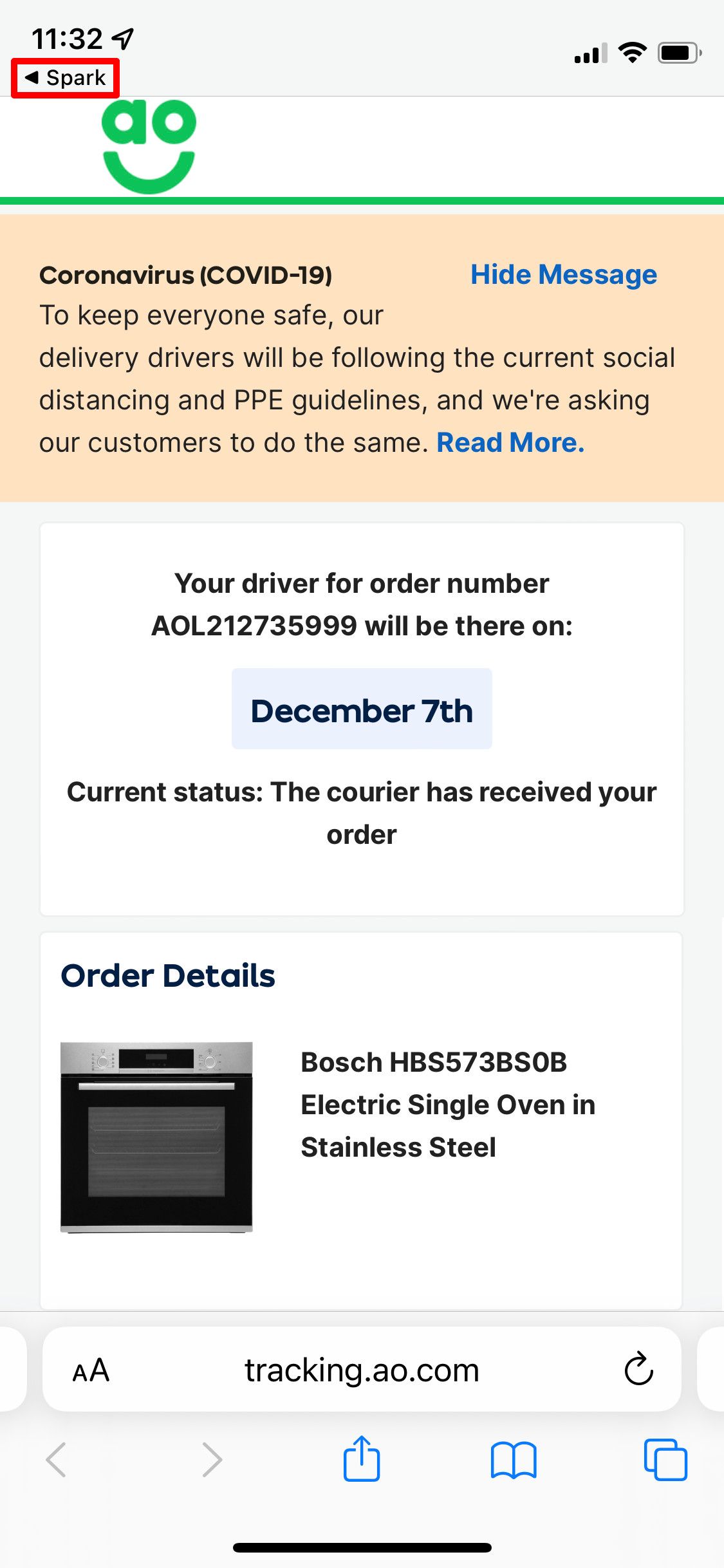A screenshot from a mobile phone displays a detailed order tracking page from the company "Spark." At the top of the screen, the date reads "11-32" (presumably indicating a time of 11:32 AM or PM). The company name "Spark" is highlighted within a red box below the time. To the right are standard icons for signal strength, Wi-Fi, and battery status.

The main screen area presents Spark's corporate logo, featuring a smiley face in green: its eyes formed by the letters 'a' and 'o' and a curved smile beneath. A notification centered at the top of the screen informs users about the company's COVID-19 safety measures, stating that their delivery drivers are adhering to social distancing and PPE guidelines. Customers are urged to do the same, with an option to read more about these policies.

Below this, there's detailed information regarding the delivery driver and the order. It mentions the driver's order number and indicates the expected delivery date, which is December 7th. The current status shows that the courier has received the order. 

Further down, the order details are specified. The item being tracked is a Bosch HBS573BSOB electric single oven in stainless steel, visualized with an accompanying image of the product showcasing its stainless steel and black design. At the bottom, a search bar labeled "tracking" suggests this screen is part of an app dedicated to tracking delivery items.